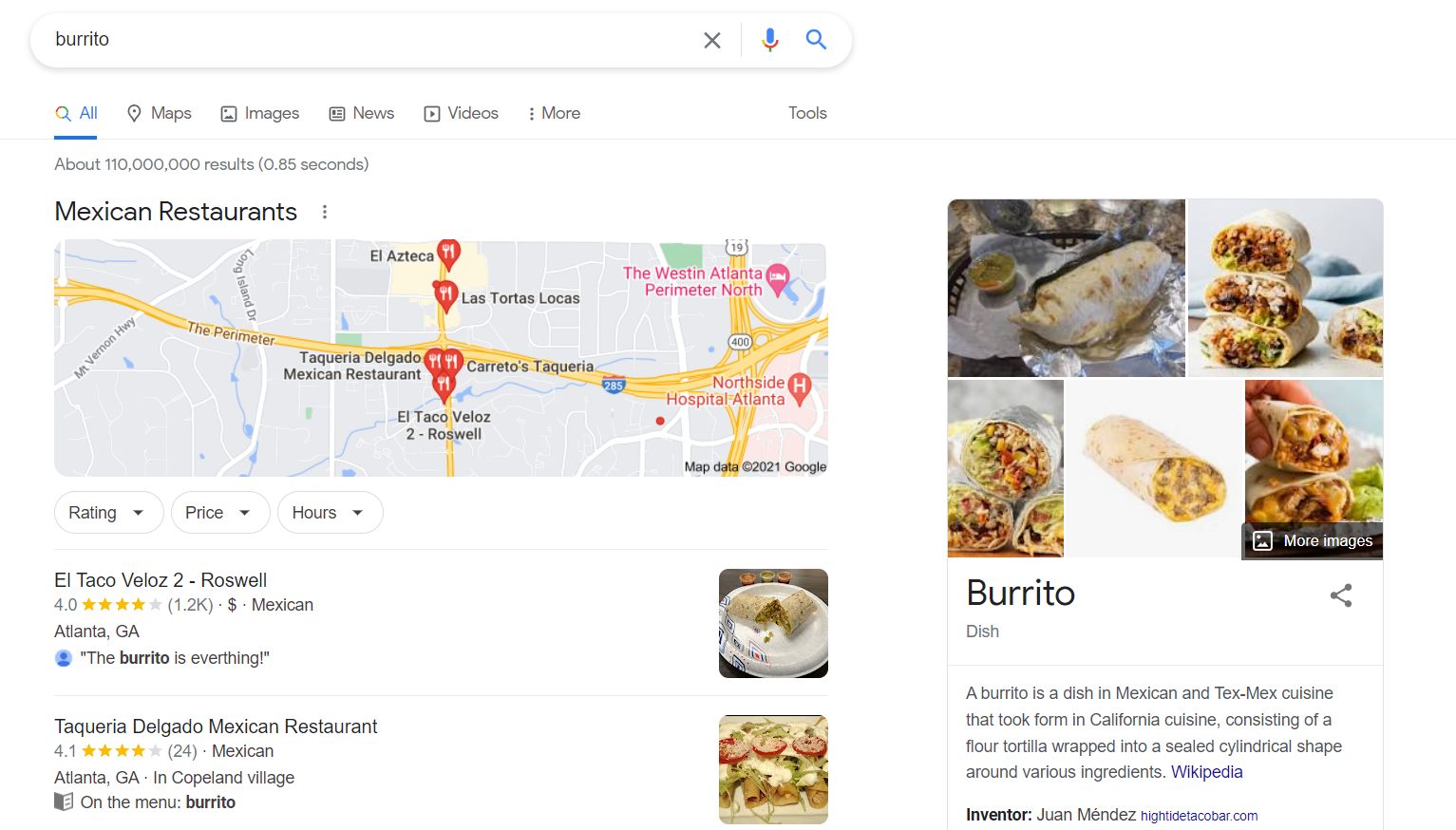This image is a screenshot of a Google search result for the term "burrito." The search results prominently feature a section highlighting local Mexican restaurants, complete with a detailed map. The map is annotated with red pin markers indicating the locations of these eateries. Major highways, bridges, and various street names are clearly visible, aiding in navigation. Within the search result, two restaurants are specifically highlighted, each boasting a four-star rating. Accompanying the listings is a vivid photograph depicting a delicious burrito, providing a visual enticement. Additionally, to the side of the main search results, there is a concise definition of what a burrito is, noting the different variations that exist for this popular dish.